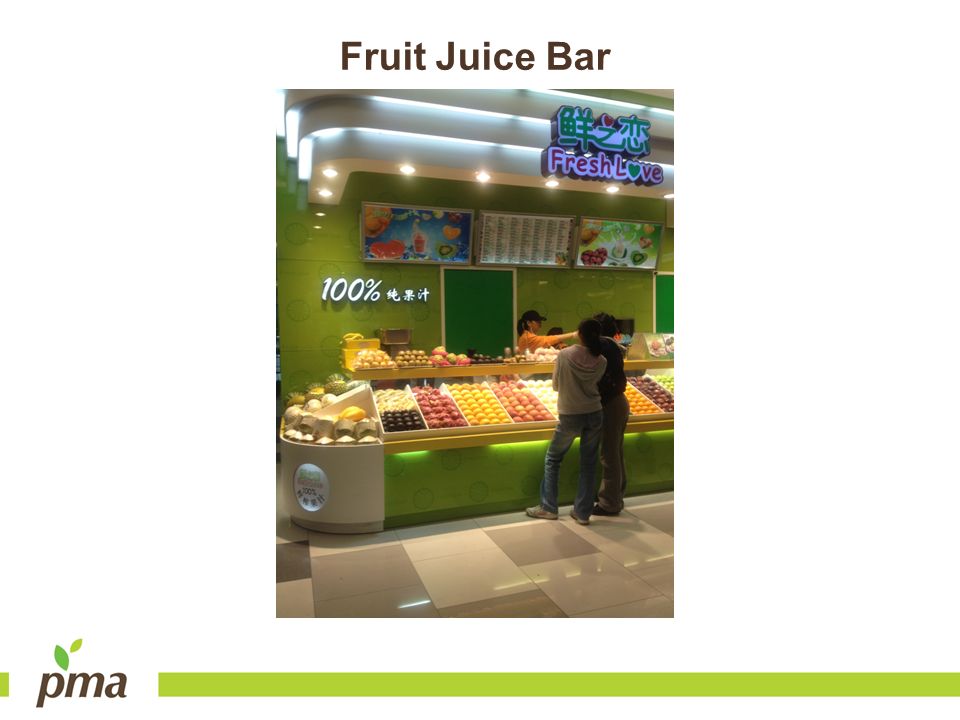The image depicts a vibrant fruit juice bar, as indicated by the title "Fruit Juice Bar" prominently displayed in a brown font against a white background at the top-center. Below the title, the bar's name, "Fresh Love," is creatively written in dark pink Comic Sans-like font, with the letter 'O' replaced by a green heart and outlined in white. There is also a possible translation in Chinese or Japanese above this title.

The storefront is predominantly decorated in shades of green and is well-lit, with lights illuminating the area from above. The bar counter is brimming with an assortment of colorful fruits including beige, brown, red, yellow, and orange varieties, neatly divided into sections. Behind the counter, a friendly employee dressed in an orange shirt and cap, with a ponytail pulled through, stands ready to assist. Above the counter are three TV screens displaying advertisements about the fruits along with a sign that brightly reads "100%"—potentially illuminated.

In front of the counter, two casually dressed people stand closely together on a shiny beige checkered tiled floor, examining the fruit options. At the bottom left of the image, the logo "PMA" is displayed alongside a long green line, adding a touch of brand identity to the scene. The overall setting is that of a clean and organized storefront, focused on promoting fresh, healthy fruit juices to customers.